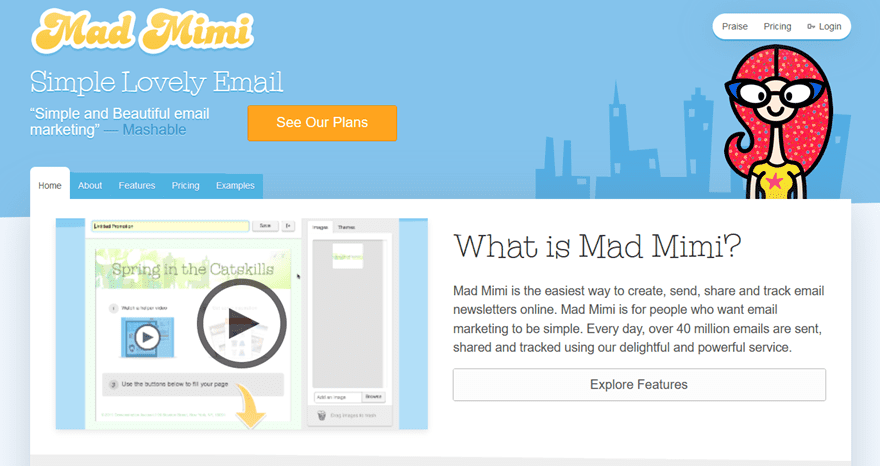This is a detailed descriptive caption for the given image:

The image is a screenshot featuring a predominantly blue background. Dominating the right side of the top half is a vector illustration of a city skyline, accompanied by a cartoon woman with bright red hair and large, cat's eye-style glasses. The woman is depicted wearing a short-sleeved yellow t-shirt adorned with a red star in the center. To the left of this illustration is the text "Mad Mimi" with a phonetic spelling below it, "M-I-M-I," followed by the tagline "Simple, lovely email. Simple and beautiful email marketing." A subtle note attributes a quote to "Mashable," and a call-to-action invites viewers to "See our plans." 

In the upper-right corner of the image, there are menu options labeled "Praise," "Pricing," and "Login." At the bottom of the image, another menu bar includes tabs for "Home" (which is currently selected), "About," "Features," "Pricing," and "Examples." 

Beneath this setup is a graphical representation of a webpage titled "Spring in the Catskills" with a prominent circular play button in the center. To the right of this representation, a text block provides an introduction to Mad Mimi: "What is Mad Mimi? Mad Mimi is the easiest way to create, send, share, and track email newsletters online. Mad Mimi is for people who want email marketing to be simple. Every day over 40 million emails are sent, shared, and tracked using our delightful and powerful service." Below this, a link invites users to "Explore Features."

Structurally, the image is wider than it is tall, with no photographic elements. The graphics are entirely illustrative, featuring no animals or automobiles.